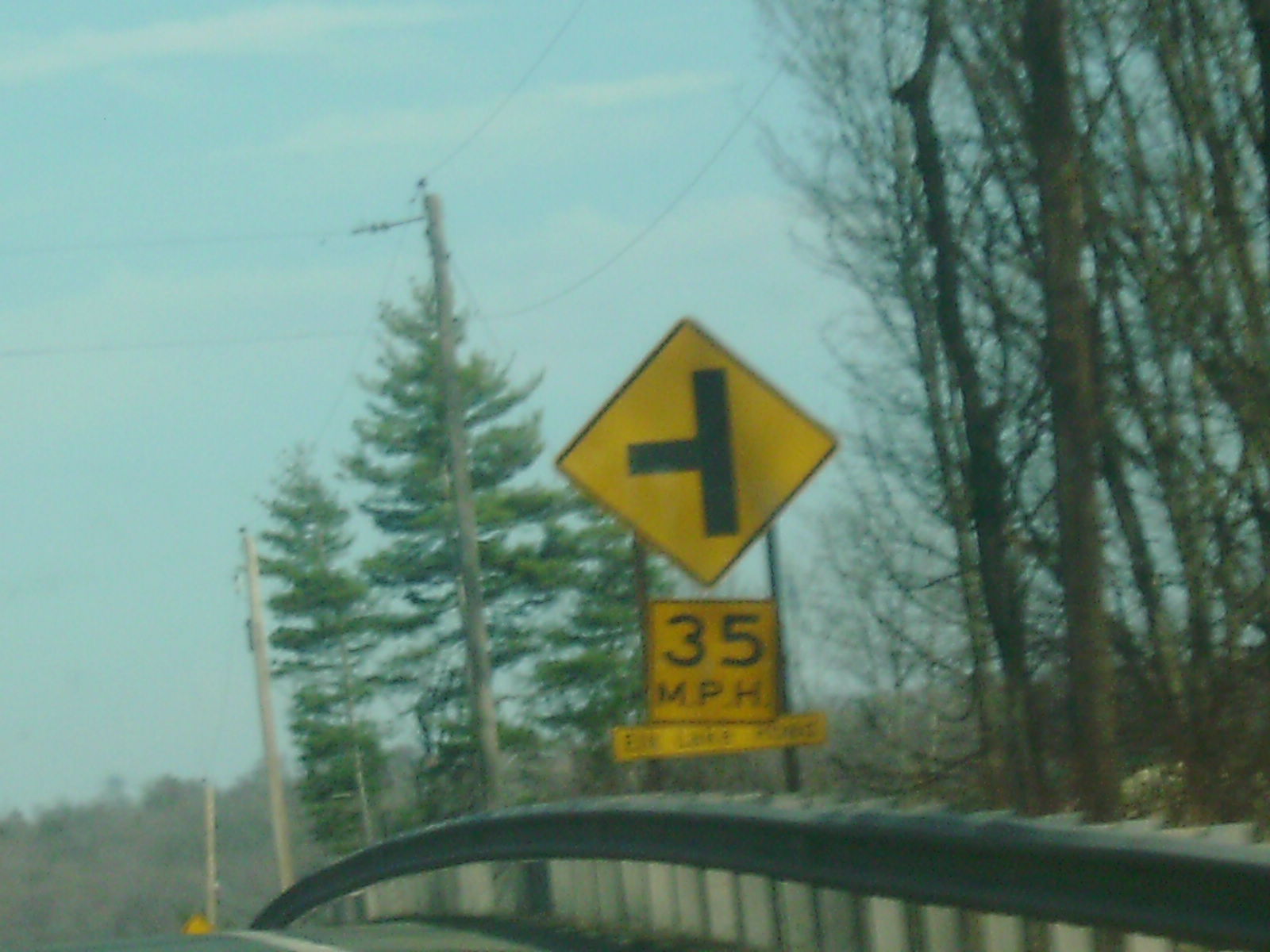The image captures a daytime scene from the passenger side of a vehicle on a road, with a clear, light blue sky occupying the upper three-fourths of the frame. A black asphalt road with a barely visible white line and a solid yellow line on the left is prominent in the foreground. On the right side, a gray metal guardrail supported by wooden posts runs along the road, starting from the corner and curving downward.

Several power poles with crossing wires are situated along the right side of the road, indicating proximity to a town or city amidst a forested area. A yellow diamond-shaped sign with a black outline warns of an upcoming T-intersection to the left. Below it, a square yellow sign displays a speed limit of 35 miles per hour in black. Farther down, another yellow sign is partially obscured, possibly indicating East Lake Drive.

The landscape includes numerous evergreen and leafless deciduous trees with visible brown trunks and branches, some towering over the horizon. In the background, a tree-covered ridge with greenery is visible, blending with the skyline seen through the thin branches of the trees.